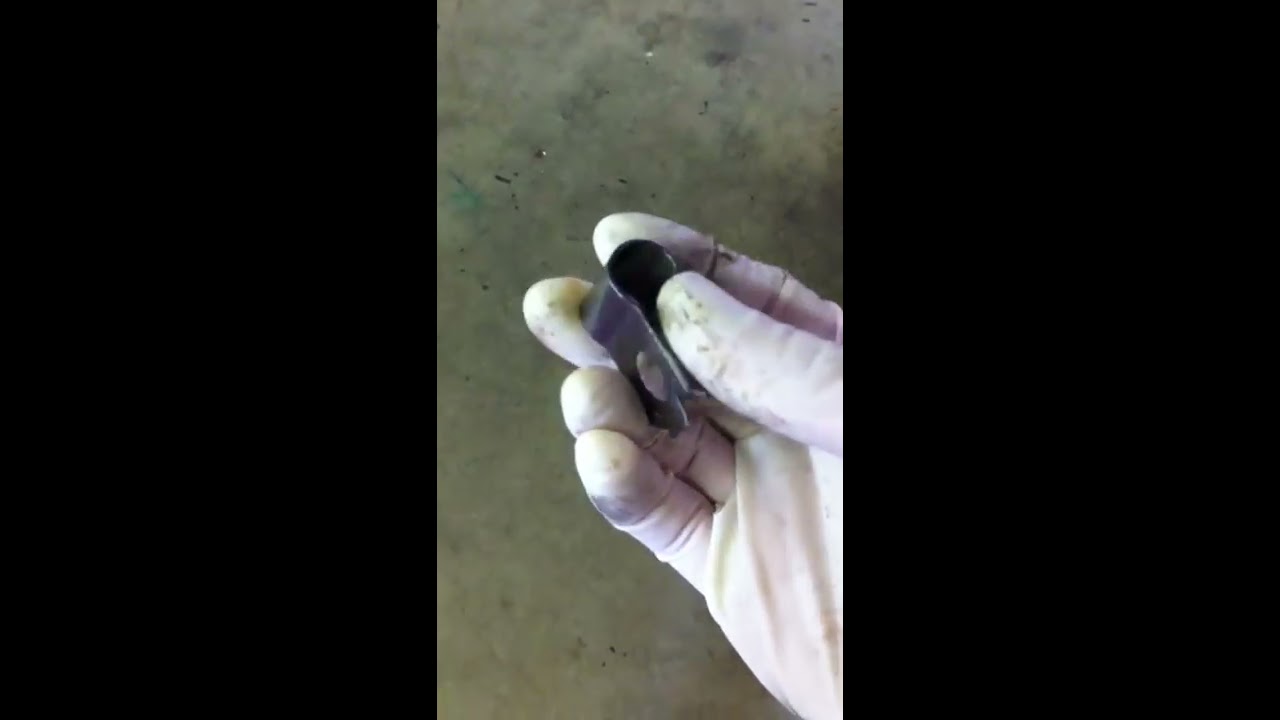The image, appearing as a still from a mobile video in portrait mode, is heavily bordered by large black bars on either side, resulting in a narrow central focus on the hand of a person. The gloved hand, featuring dirty and green-stained white latex gloves, holds a small black metallic piece, which is curved and appears to have broken off from something larger. This piece is positioned between the person's thumb, forefinger, and middle finger. The person stands over a floor that looks like rocky concrete, possibly within a garage, with some debris scattered around. The overall tone of the image highlights the close-up on the hand, giving the impression of a detailed and focused examination of the held object amidst a backdrop that is difficult to discern, potentially a dirty green surface or cement.